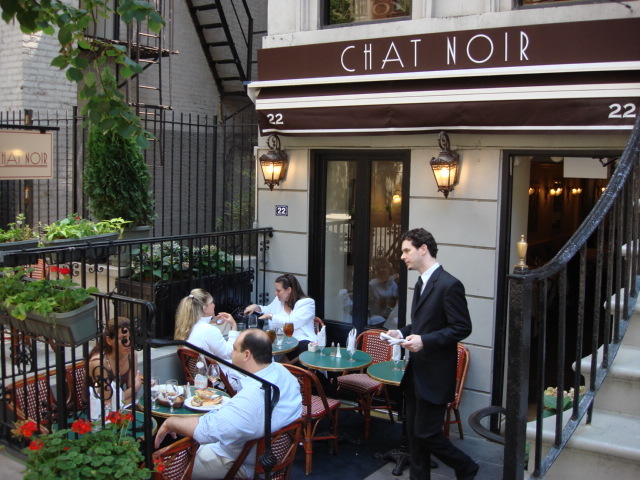The image features the words "Chat Noir," which translates to "Black Cat" in French, displayed in white, all-capital, sans-serif font. This text is set against a brown-colored strip or background. Flanking this brown strip, the numbers "22" appear on both sides. Decorative lanterns or lamps hang on either side of a black-framed window situated on the wall behind the "Chat Noir" sign. In the bottom right corner, a black stairwell is visible, appearing to lead to an upper level of the building.